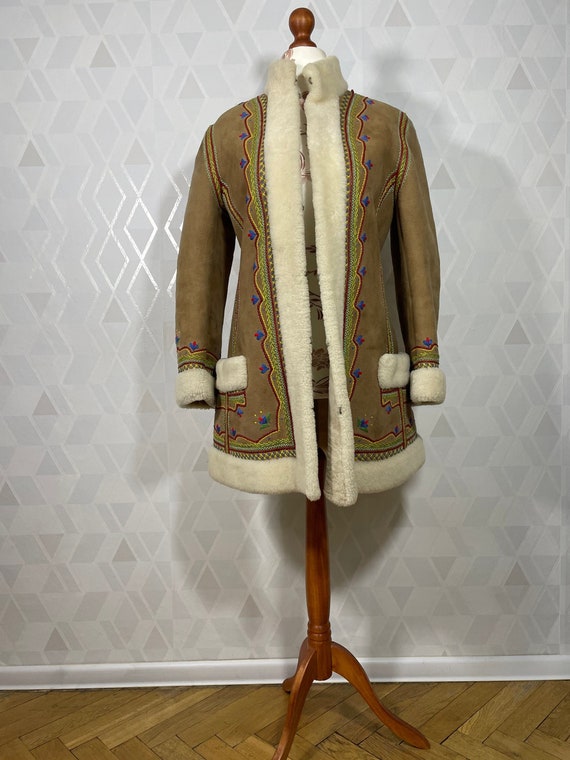This image features a vertical wooden coat rack standing on a wooden parquet floor, against a light silver wall adorned with a reflective diamond pattern. The rack, darker brown with an orangish hue and supported by three legs, holds an elegant tan women's winter coat. The coat boasts a fur lining along the front, bottom edge, sleeve cuffs, and pockets, enhancing both its warmth and style. Detailed stitching in green, red, and blue decorates the front, while small purple shapes, reminiscent of buttons, add a subtle, decorative touch. The overall design evokes a blend of fashionable and practical, making it ideal for cold climates. The scene is well-illuminated, casting shadows that emphasize the textural contrasts between the coat, the wooden flooring, and the glimmering wall behind.